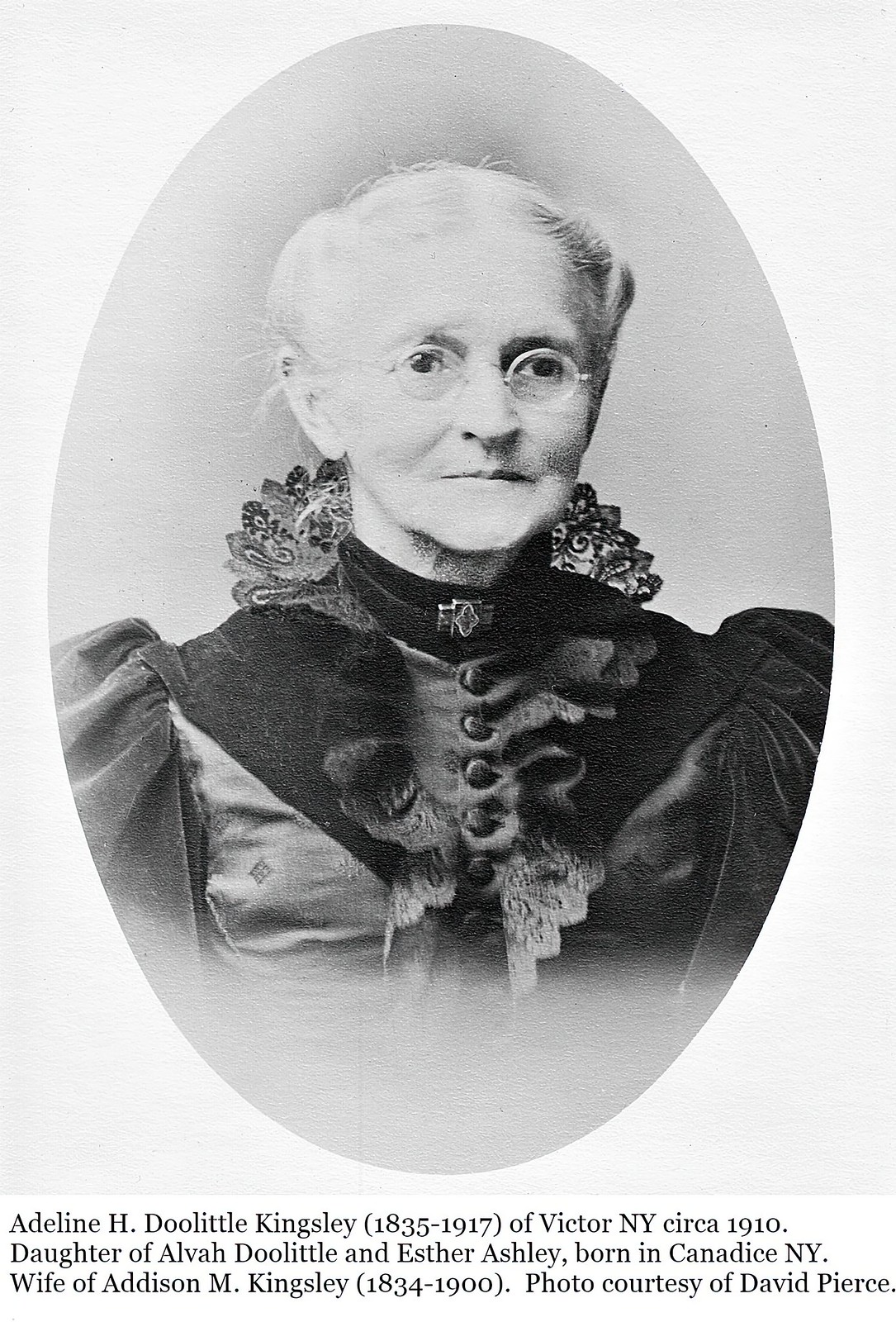The black and white portrait features Adeline H. Doolittle Kingsley (1835-1917) from Victor, New York, circa 1910. Adeline, the daughter of Alva Doolittle and Esther Ashley, and wife of Addison M. Kingsley (1834-1900), is depicted as an elderly woman in her 60s or 70s. She is wearing 19th-century attire, specifically a Victorian-style black dress with prominent fluffy, puffed shoulders and multiple buttons down the front. A decorative pin adorns her collar, resembling a cross with an additional symbol. Adeline, who has short hair and glasses, appears to be smirking slightly. The photo is egg-shaped and set against a white background, with the credit "Photo courtesy of David Pierce" below. This scanned image preserves the historical essence of Adeline in the early 20th century, showcasing her dignified and somewhat stern demeanor.